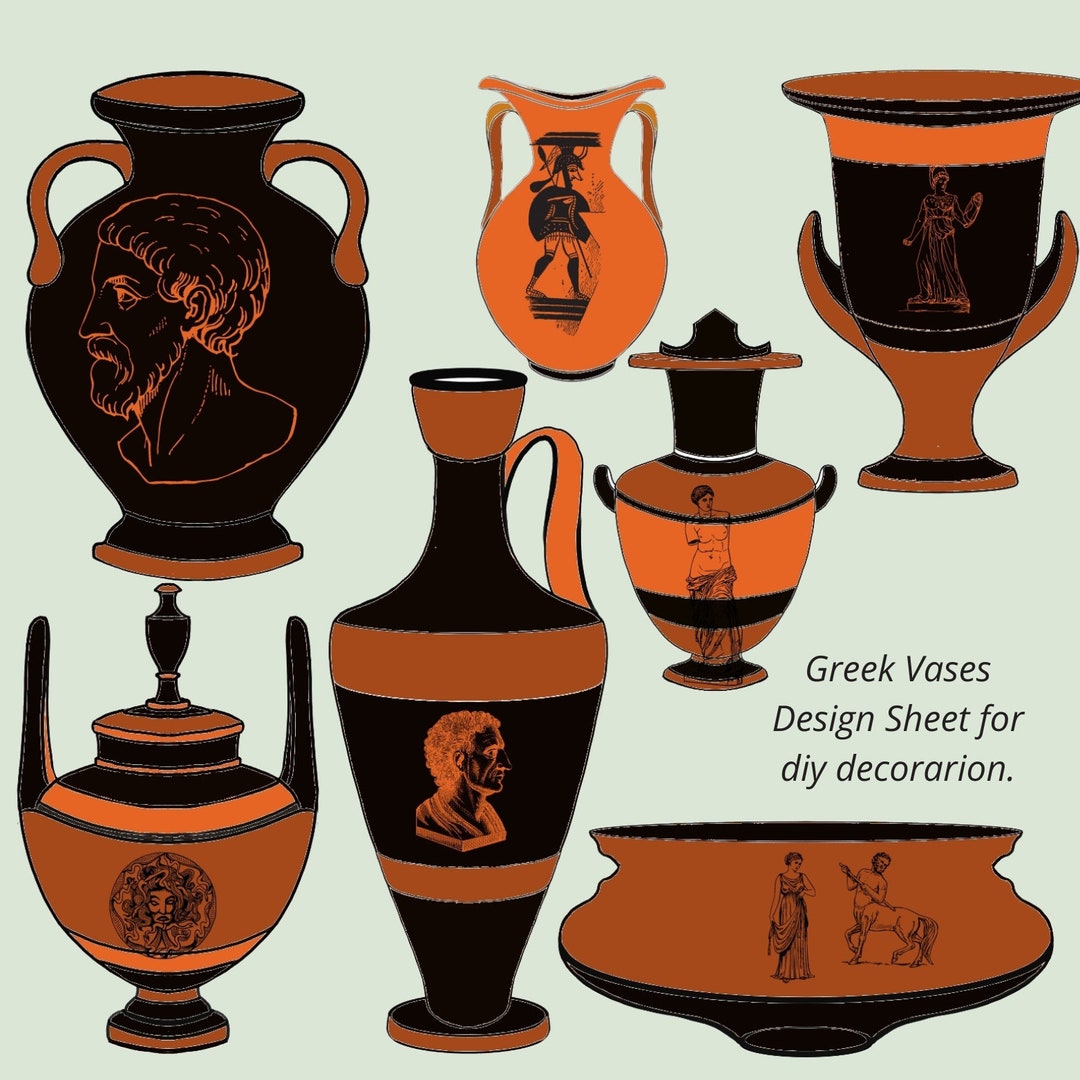The image is of a Greek Vases Design Sheet for DIY Decoration against a light green background. It features a collection of vases in varying sizes and shades of orange and black. Among the vases, there is a prominent large black vase with two handles on each side. The vases are adorned with intricate drawings, including ancient Greek figures, mythological scenes such as Zeus and a centaur, and busts of historical characters. Some vases depict full-bodied figures, while others highlight specific Greek statues. The variety in their designs and the detailed artwork suggest these vases could also be functional for holding drinks. The image is captioned towards the bottom right with "Greek Vases Design Sheet for DIY Decoration," indicating its purpose for creative projects.